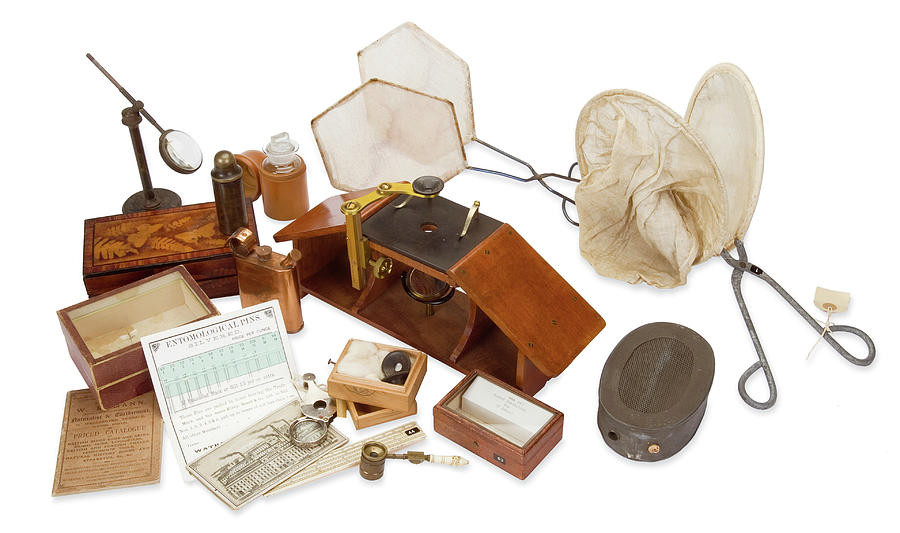The image depicts an antique insect or butterfly capturing, examining, and mounting kit laid out against a white background. The kit includes two large, scissor-like structures with circular netted areas, reminiscent of strainers, positioned in the upper center to the upper right portion of the image. A magnifying glass mounted on a swivel stand, allowing for easy adjustment, is prominently featured. Several small wooden boxes, intricately decorated with wood-burned leaf and insect designs on their lids, are spread across the scene. At the center, an examination structure resembling a tent consists of two solid slanted wooden side pieces and multiple compartments underneath. Additionally, there are various boxes containing different types of lenses and eyepieces. One box has a card leaning against it that reads "endomorphological pins."